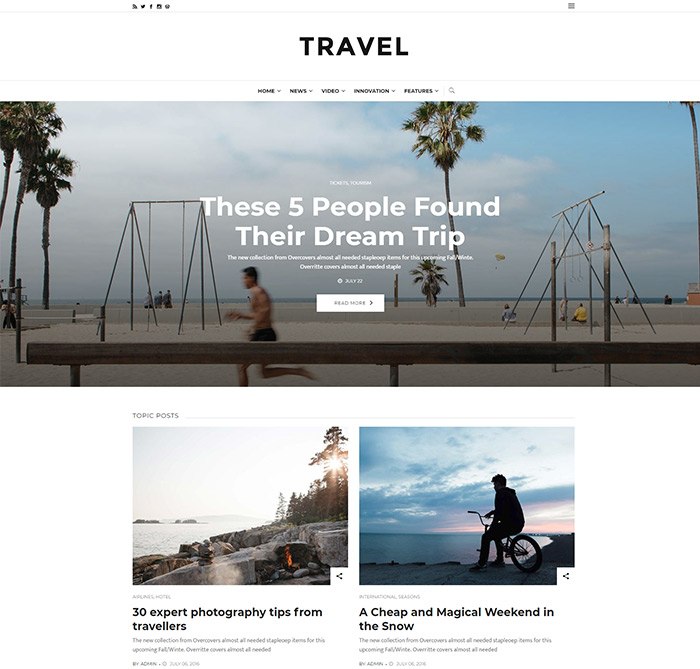The top portion of the image features a white background with the word "TRAVEL" prominently displayed in black, bold, capital letters. Beneath this header, a black navigation bar lists categories: Home, News, Video, Innovation, and Features. 

The main background image presents a picturesque beach scene. On the sandy shore, a man can be seen running and placing poles into the ground. The scene is adorned with four tall palm trees—three on the left and one on the right—with a smaller fifth palm tree nestled amongst them. To the left, a swing set is visible, while the right side of the playground features monkey bars. The vibrant beach setting is accentuated by a yellow kite soaring in the sky, framed by the expanse of the ocean and a clear, bright sky above.

In white text overlaying the beach image, the caption reads: "These five people found their dream trip." Below this, a smaller text snippet in black mentions, "Where's the new collection from?" 

Towards the bottom of the image, a white rectangular box contains the call-to-action "Read More" in black text. The lower left corner of the image displays "Topic Post" in gray, with the caption, "30 Expert Photography Tips from Travelers," in bold black text. Further down, a partially obscured line reads, "The new collection from," with the rest of the text indecipherable.

On the right side, another bold black caption reads "A Cheap and Magical Weekend in the Snow," with additional text below that blurs into unreadability. The captions in larger, bold black text stand out against the otherwise smaller and less distinct text elements.